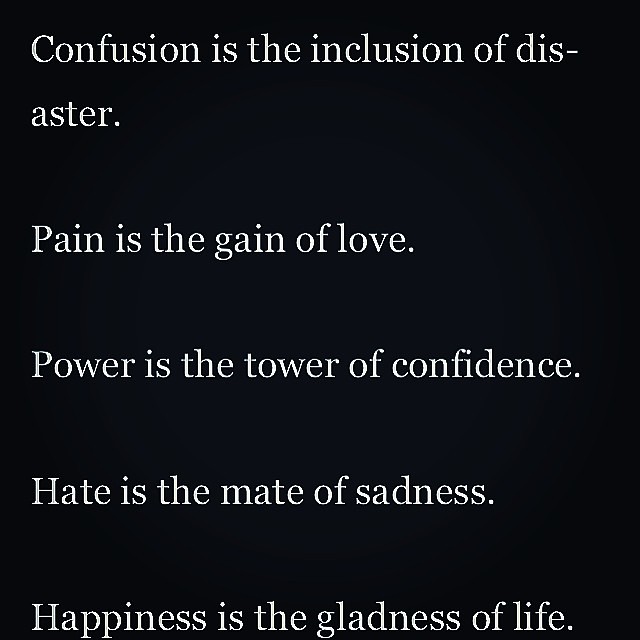The image is a simple yet striking typography graphic design in a square format, designed to convey an inspirational message. Set against a completely black background, the white serif text consists of five thought-provoking statements: "Confusion is the inclusion of disaster. Pain is the gain of love. Power is the tower of confidence. Hate is the mate of sadness. Happiness is the gladness of life." Each sentence is carefully aligned to the left, with sufficient space between lines for easy reading. The style resembles a motivational message often found on social media platforms like Pinterest, utilizing a clean and minimalist design reminiscent of Times New Roman font. Notably, the first sentence spans two lines, breaking the word "disaster" into "dis-aster," while the remaining sentences fit on single lines. The overall design is simple and impactful, embodying the essence of digital typography art.